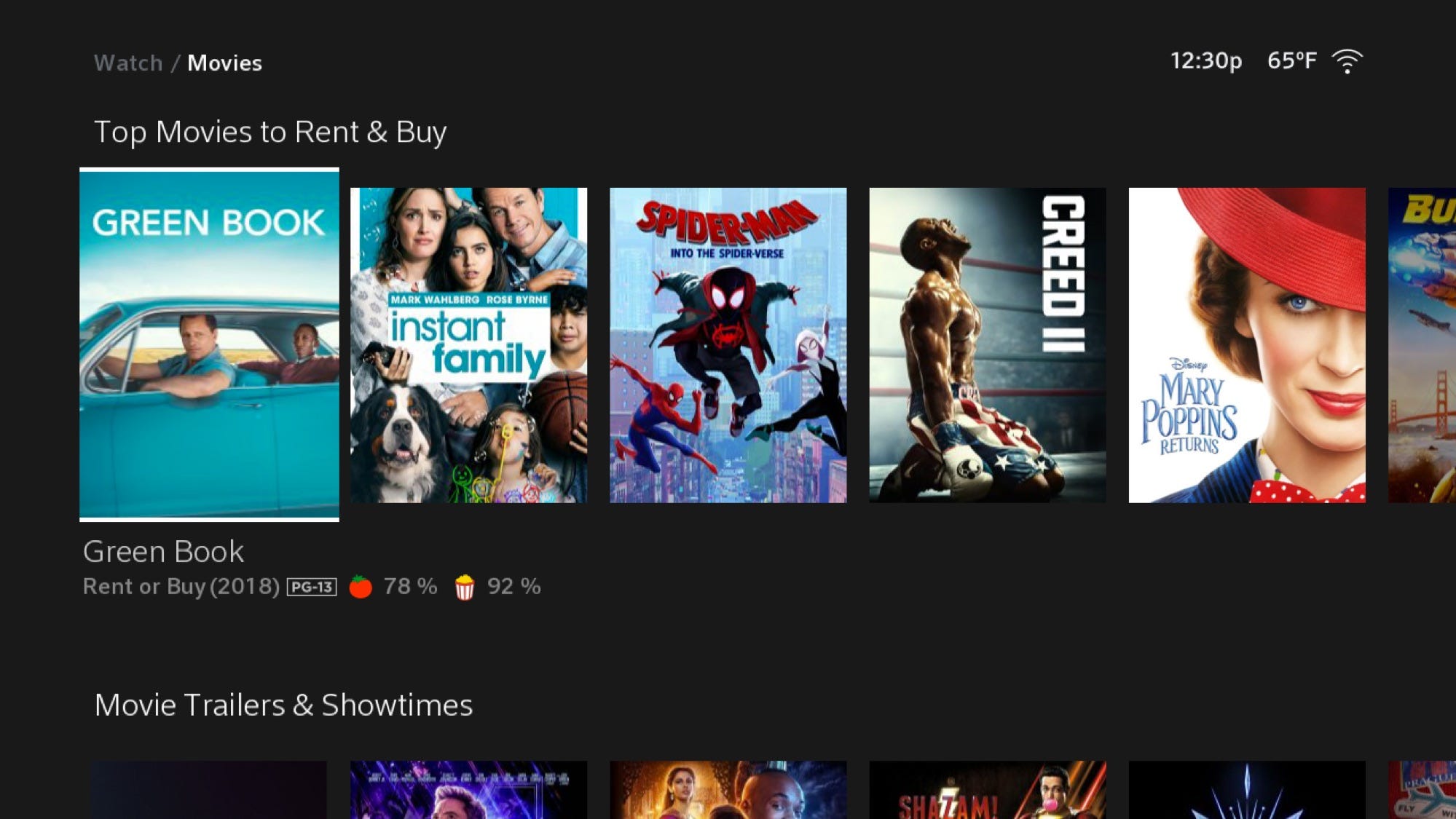The image captures a screenshot from an unidentified video streaming application, possibly Amazon Prime Video, likely viewed on a tablet, perhaps a Fire tablet based on the orientation and screen size. The focus of the screenshot is on the "Top Movies to Rent and Buy" section, prominently displaying titles like "Green Book," "Instant Family," "Spider-Man: Into the Spider-Verse," "Creed II," and "Mary Poppins Returns," all of which are relatively recent releases. The highlighted movie, "Green Book," shows detailed information including its PG-13 rating, a Rotten Tomatoes score of 78%, and a user rating of 92%. The lower part of the image glimpses a partially visible section dedicated to "Movie Trailers and Showtimes," indicating that the full interface offers a variety of movie-related content.